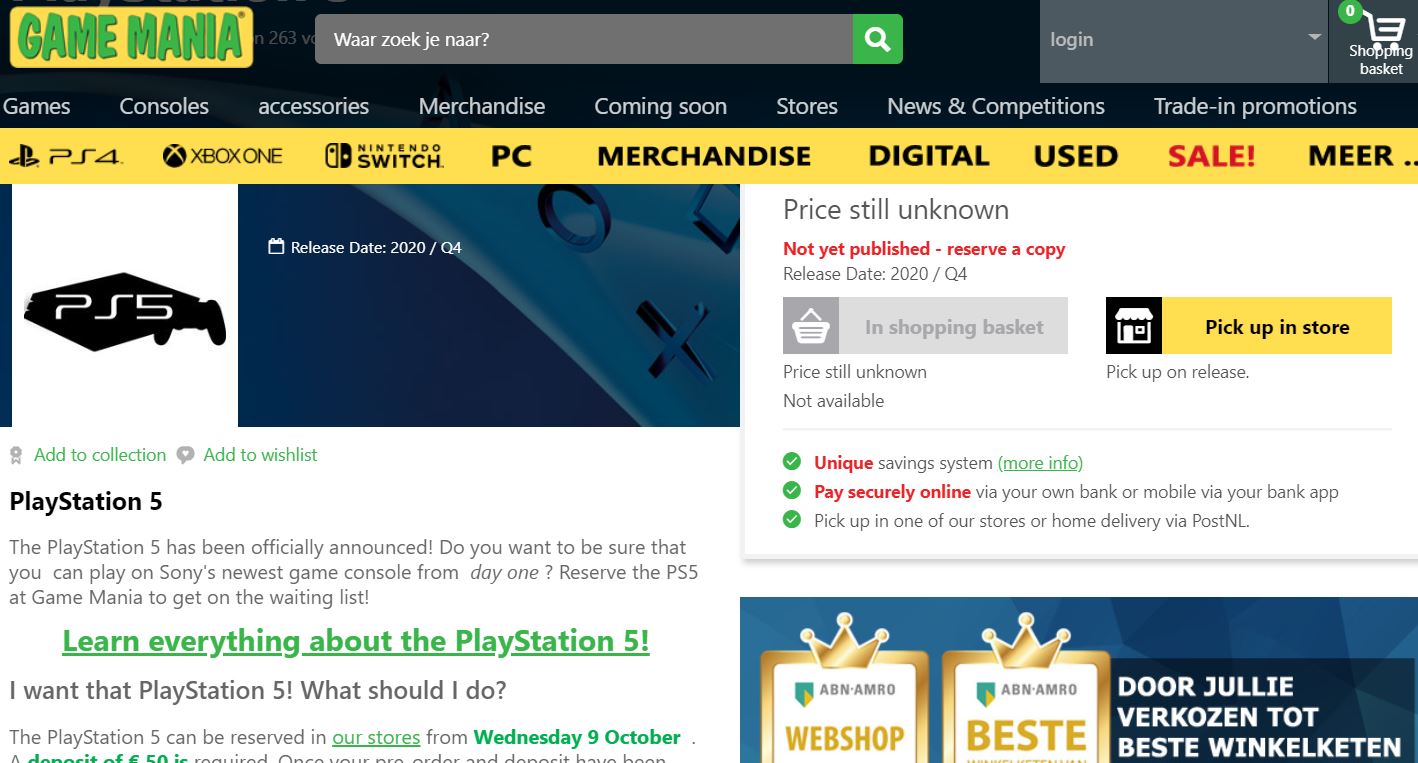**Detailed Caption:**

This image captures a detailed screenshot of a website's home page dedicated to shopping for video games. The top portion features a black border approximately two inches in height. In the top left corner, there is a striking yellow rectangle with "Game Mania" inscribed in green text.

Beneath this, a gray search bar spans halfway across the page, containing the placeholder text "WAARCOEKJENAAR?" in white. To the right of the search bar, a green square with a white search icon is positioned.

Adjacent to the search bar on the right, a gray tab allows users to log in, with a white shopping basket icon next to it displaying a green zero above a white zero, indicating the current number of items in the cart.

Immediately below these elements, a navigation menu in white text runs horizontally across the screen. It includes categories such as "Games," "Consoles," "Accessories," "Merchandise," "Coming Soon," "Stores," "News and Competitions," and "Trading Promotions."

A yellow tab below the navigation menu highlights various gaming platforms: "PlayStation 4," "Xbox One," and "Nintendo Switch," each accompanied by respective icons. Additional categories follow, including "PC," "Merchandise," "Digital," "Used," "Sale" (in red), and "MEER..." with ellipses indicating more options.

On the right side of the page, a small promotional photo displays a blue background with a partial image of a PlayStation controller in the top right corner. Below the image, black text reads "PlayStation 5," followed by a descriptive paragraph about the console. Green, bolded, and underlined text invites users to "Learn everything about the PlayStation 5." Additional information lines are included, with black text indicating "Price still unknown." Adjacent to this, yellow and red text states "Not yet published - reserve a copy." There is a gray tab provided for adding the item to the shopping basket, and a yellow tab indicating the option to "pick up in store" in black text.

Beneath these sections, three green circles with white checkmarks are vertically aligned, each accompanied by a line of informational text. Finally, a small pop-up tab at the bottom of the page, displayed in German, is visible—though its content remains unspecified.